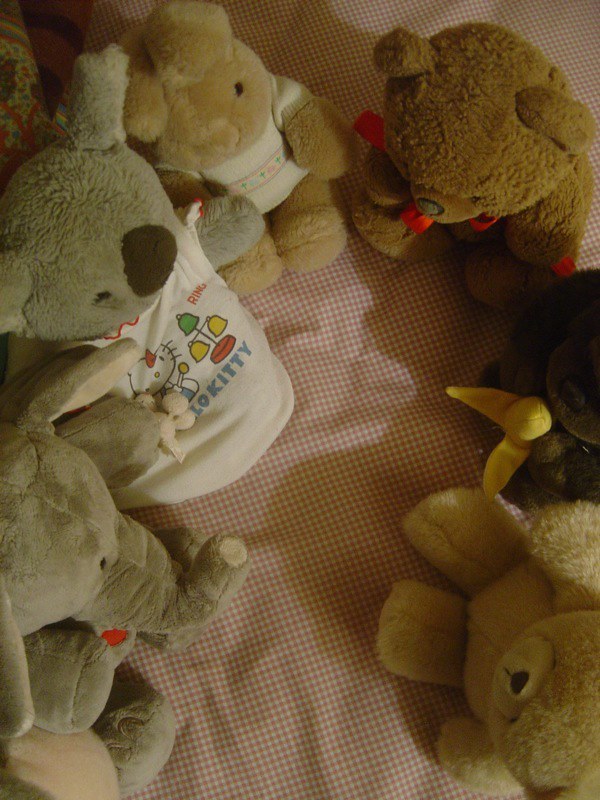In a cozy child's bedroom, a pink and white checked blanket is spread out, forming the setting for a delightful tea party with an endearing assembly of stuffed animals. In a semi-circle across the blanket sit a variety of plush friends, each with unique characteristics and charming details.

At the bottom right-hand corner is a gray elephant, its trunk pointed upwards, adorned with a little red heart beneath its tusk. Its floppy ears have pink interiors, and it sits with its arms outstretched, adding to its inviting appearance. Adjacent to the elephant is a fluffy koala bear, comfortably seated and dressed in an adorable Hello Kitty shirt decorated with the iconic white cat, a red bow, a cap, blue overalls, and colorful bells with the word "ring" printed on it. In the middle sits a brown rabbit wearing a pink sweater adorned with pink and blue flowers in a band across it. The rabbit's ears are turned downward, and it has black eyes and outstretched arms, giving it a serene demeanor.

Next to the rabbit is a well-loved brown teddy bear, distinguished by a big red bow around its neck and a black nose that shows signs of affection, with its fur worn off on its foot from many hugs. To its left is a gorilla intently eating a peeled banana, completing a whimsical touch to the gathering. Finally, in the bottom left-hand corner, there is a tan bear sitting with its arms outstretched.

All the animals are arranged on the checked blanket, seemingly gazing at each other, creating a warm and inviting scene. The details of their clothes and positions suggest a snapshot taken from above, capturing this charming gathering of fluffy friends as they await their child's return to join the fun.